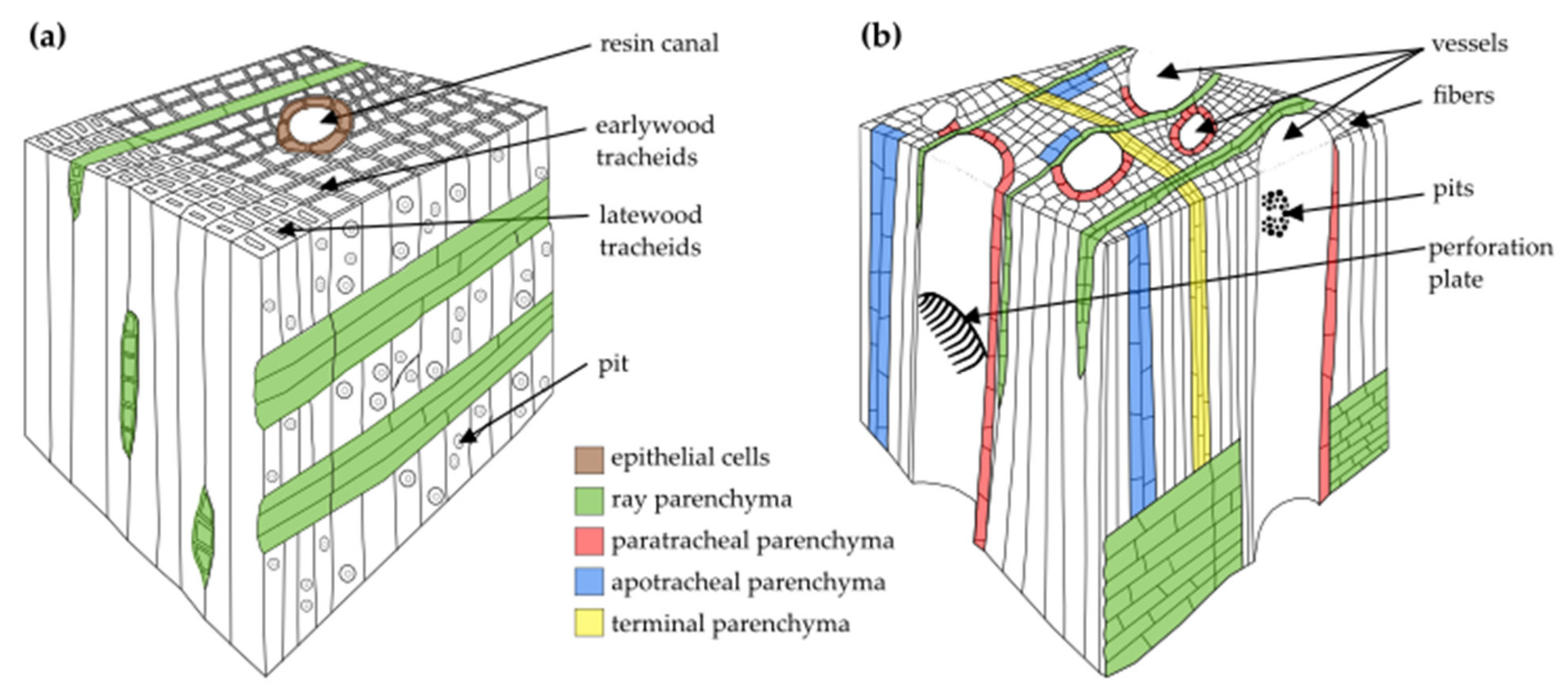The image features two diagrammatic cubes, labeled A and B, each illustrating different cellular structures, possibly of wood or similar fibrous material. Cube A is white with vertical and horizontal striped patterns on its sides and a grid pattern on top. Marked with green-colored labels, arrows point to features such as resin canal, early wood tracheids, late wood tracheids, and pit. A color-coded legend at the bottom identifies various cell types, denoted by five distinct color codes, although some specific terms are hard to pronounce. Cube B, slightly wavy and also lined horizontally and vertically with a similar grid top, includes markings in blue, green, red, and yellow. Its labels, pointed out by arrows, identify vessels, fibers, pits, and a perforation plate. A central legend explains the color codes for each cube. Both cubes detail different cellular components, providing a comparative visual representation, albeit without explicit information about the overall context of the diagrams.